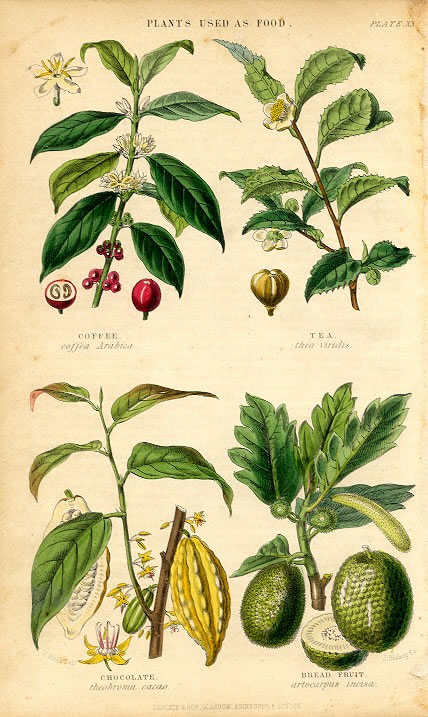The image is a detailed botanical illustration of four different plants used as food, presented on a slightly yellowed or off-white page resembling a booklet or pamphlet. The title at the top reads "PLANTS USED AS FOOD" in black, capitalized text. Each plant is meticulously drawn, showing various parts like stems, leaves, flowers, and the final products. The plants are arranged in two rows and two columns.

In the top left is the Coffee plant, identified as Coffea arabica. The illustration features a branch with clusters of red coffee berries at different stages of growth, along with broad green leaves.

The top right showcases the Tea plant, noted as Camellia sinensis. The depiction includes white flowers and green leaves, characteristic of tea plants.

The bottom left displays the Chocolate plant, Theobroma cacao. It highlights a large yellow cacao pod and a smaller green pod, which house the cacao beans, along with the leafy branches.

At the bottom right is the Breadfruit plant, categorized as Artocarpus altilis. The image includes a cut-open green breadfruit showing its detailed texture, alongside the depiction of green leafy branches.

The illustrations are primarily green but include other colors like red for the coffee berries, white for the tea flowers, yellow for the cacao pod, and varying shades of green for the breadfruit. This rich and informative layout provides insight into the botanical aspects of these edible plants.